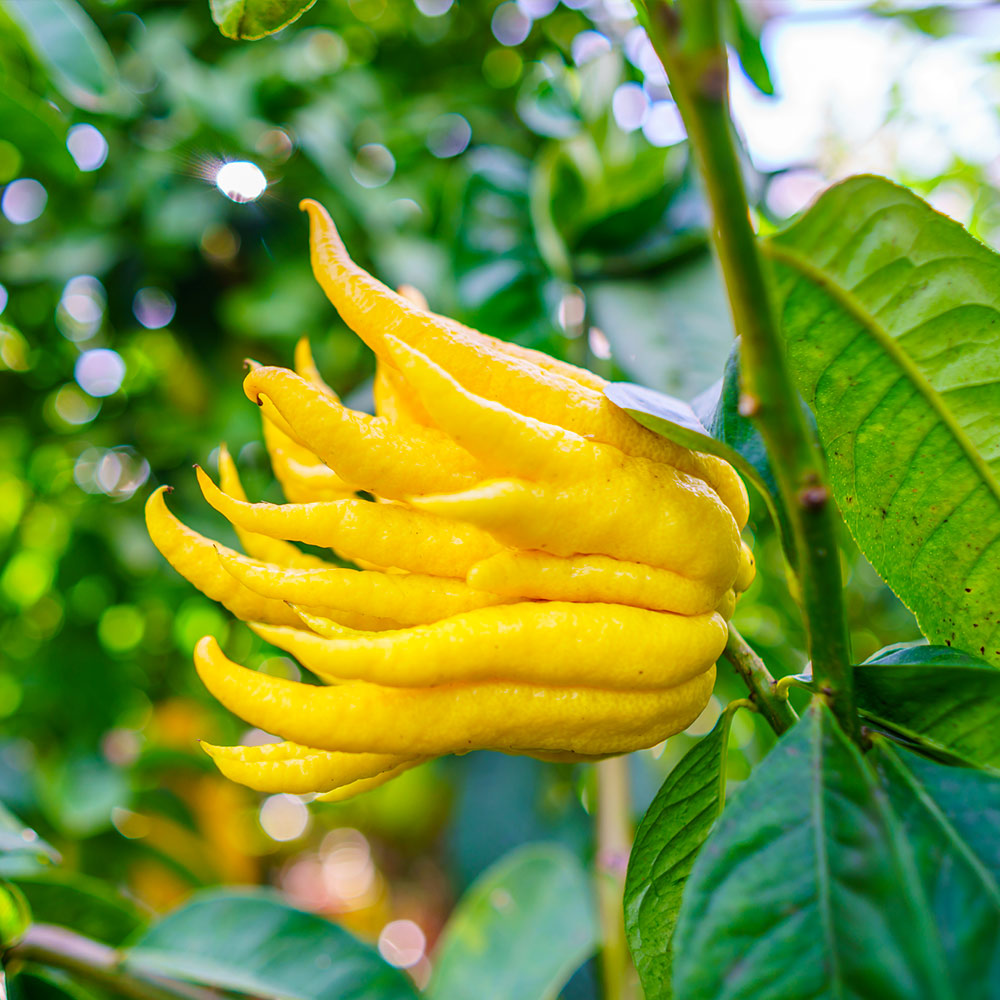This is a close-up photograph of a Buddha's hand plant, also known as the fingered citron fruit tree. The tree features thick, bright green branches and spear-shaped, glossy green leaves. The primary focus of the image is on the unique yellow fruit that resembles a bunch of small yellow fingers or carrots, with tips that hang or extend outward, creating an appearance akin to a cluster of flower petals. The texture of the fruit has a shiny, almost plastic-like quality, similar to that of a lemon. The background, slightly out of focus, showcases more greenery and hints of the blue sky, with bright green trees and white spots, contributing to the composition's depth and contrast.